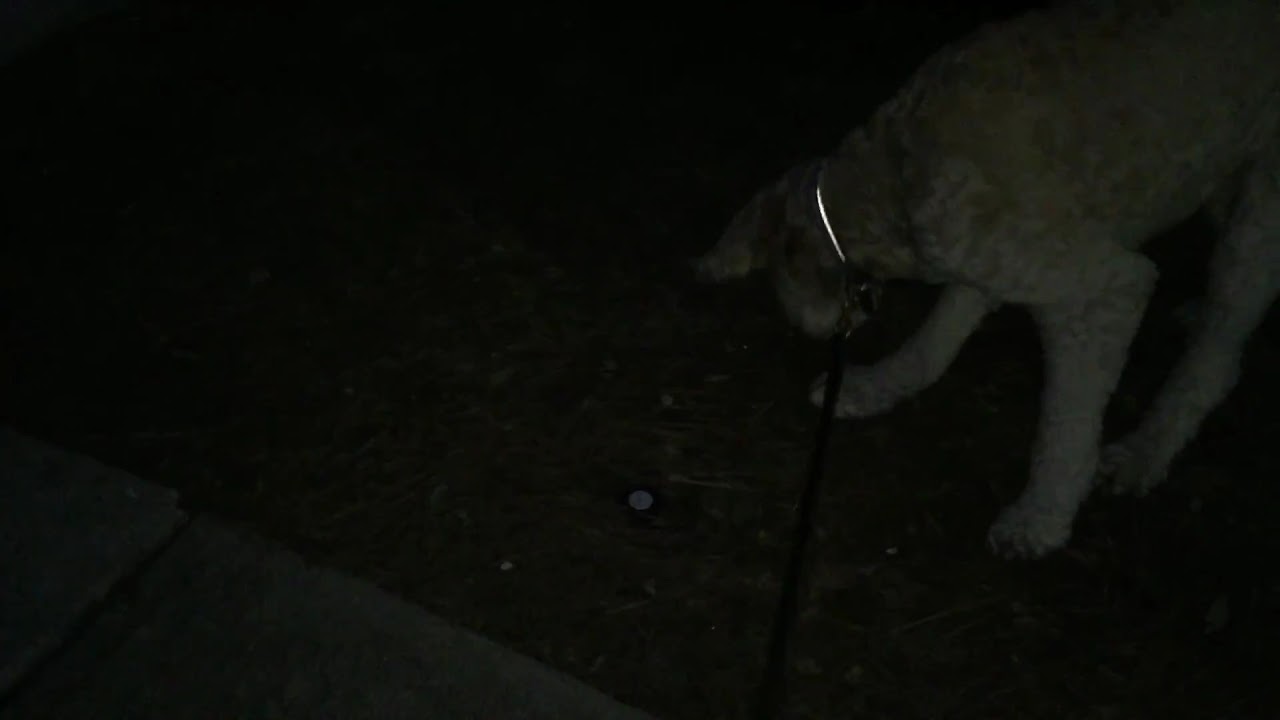This image depicts a medium-sized white dog with fuzzy fur, standing out vividly against an overall dark background. The setting appears to be nighttime, either in a backyard or on the street, with minimal lighting making it difficult to see finer details. The dog, clearly visible due to its white coat, is engrossed in sniffing the ground, possibly searching for something. It is wearing a collar attached to a black leash, though the leash’s color may be influenced by the dim lighting. Positioned to the right of the frame, the rear part of the dog is cut off, while on the left side of the image, there is a faint outline of a stone walkway. There are no additional elements such as humans, other animals, or text present in the scene.